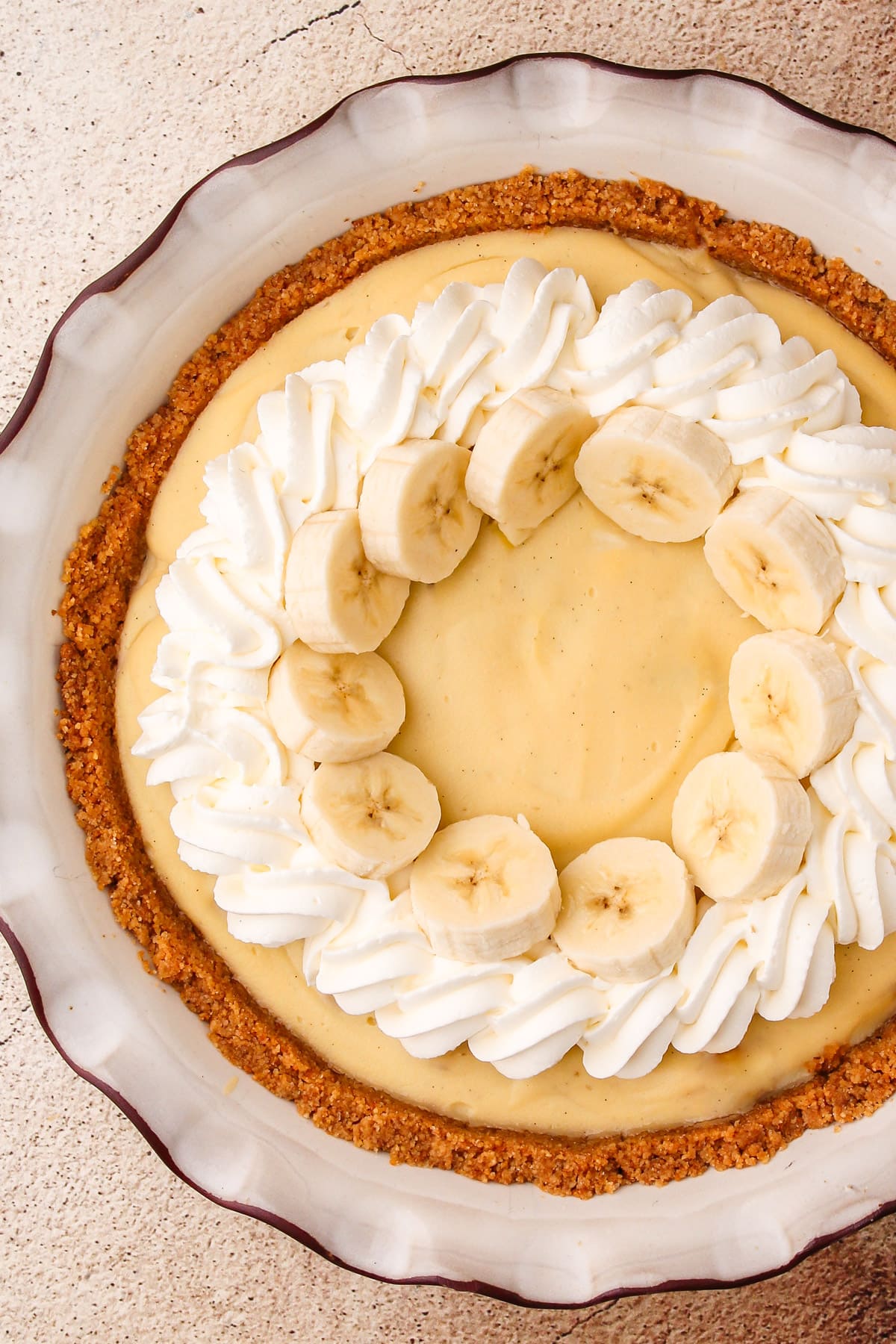This is a detailed top-down photograph of a homemade banana cream pie, showcasing its meticulous preparation. The pie features a creamy, banana-colored filling with a circular arrangement of banana slices at the center. Surrounding these slices is an artfully swirled ring of whipped cream, which has lines and designs indicative of careful application. The pie is set in a thick, brown graham cracker crust, giving it a rich, textured border. The ornate pie plate, with its ruffled and dimpled edges, has a white interior and a darker, perhaps brown, glaze along the rim and possibly at the bottom. This plate rests on a beige surface that appears to be a coarse-textured countertop or concrete floor, suggesting a natural, realistic setting. The entire uncut pie is presented in natural lighting, amplifying its homemade charm.